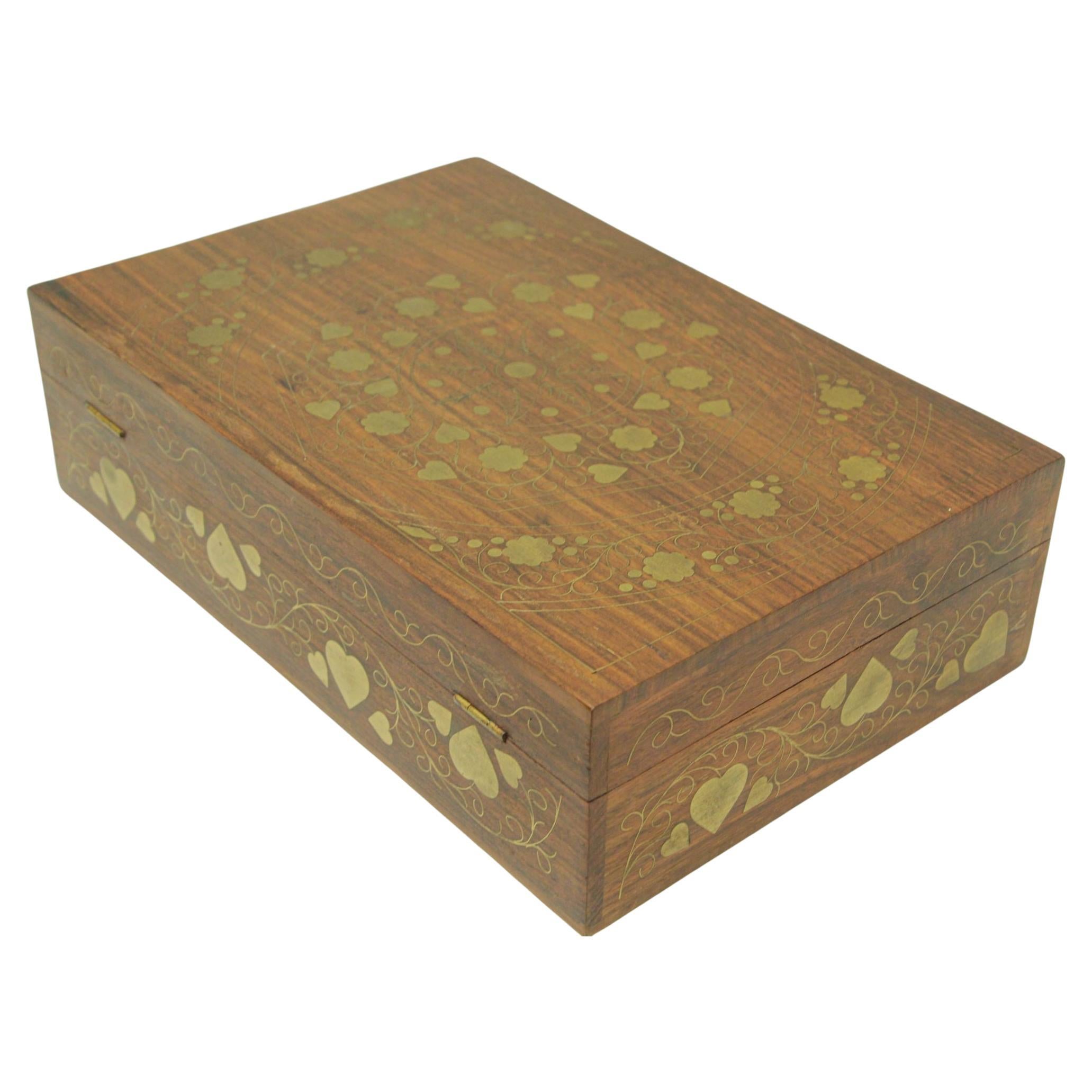The image depicts an antique wooden jewelry box, likely made from cedar wood, adorned with intricate inlay designs. The box features a rich brown hue, showcasing varying wood grains and aged with time to give an antique look. The intricate inlays consist of heart patterns that wrap around the edges of the box, rendered in an ivory or once-white material that now carries an aged, golden tint. The top of the box is elaborately decorated with a circular pattern that narrows towards the center, culminating in a single detailed flower design. Additional elements, such as delicate vines, interlace with both the hearts and flowers, adding to the overall elegance of the design. The box has small brass hinges on the left side, suggesting that the lid can be opened like a book. The entire scene is set against a clean, white background, emphasizing the ornate craftsmanship of the wooden jewelry box.